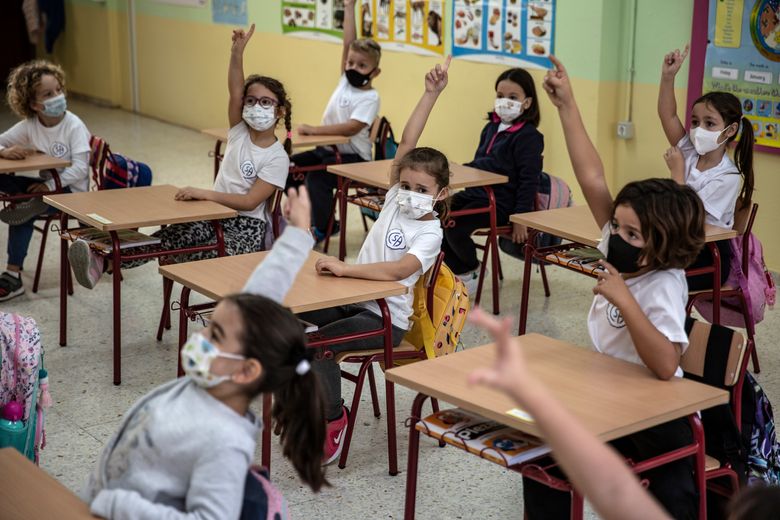This wide rectangular photograph captures a vibrant elementary classroom scene. There are three rows of desks: the furthest row starts in the middle on the right and extends diagonally upwards, the middle row begins at the bottom right corner and progresses diagonally left, and the front row is partially visible in the bottom left. The desks, constructed with red metal frames and light brown wooden tops, are paired with matching chairs featuring wooden seats and backrests. Each chair has a backpack hanging from its backrest.

The young children, who appear to be around six years old, are seated at these desks. They are all wearing white t-shirts adorned with blue logos and face masks—predominantly white, with one child donning a black mask. Many of the children's feet dangle above the floor, underscoring their tender age. In the furthest row, there are at least three students visible, four students occupy the middle row, and only a part of one child and an arm are evident in the cropped front row. Most of the students are raising their right hands with fingers pointing upwards, except for two: the middle child in the back row and a boy on the far left of the middle row.

The backdrop features a yellow and green wall adorned with several posters, though only their bottoms and some indistinguishable images can be seen. This detailed depiction highlights a typical day in the life of these enthusiastic, mask-wearing young learners amidst a bright and organized learning environment.